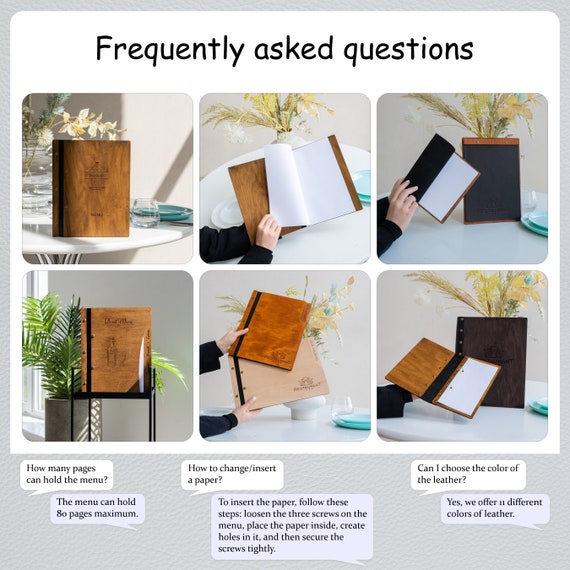The image is a detailed section from a webpage titled "Frequently Asked Questions" in black text at the top. Underneath, there is a grid of six photographs displayed in two rows of three. These photos showcase a brown notebook, which has a wooden texture, in various contexts:

1. The first photo shows the notebook standing upright on a white table.
2. The second image captures someone holding the notebook open, flipping through the pages.
3. The third photo also features an individual interacting with the notebook.
4. The fourth image on the second row highlights the notebook with a distinctive concave ridge on the right side.
5. The fifth photo compares two different styles or colors of the notebook.
6. The final image shows a dark-hued notebook in the background, and a person holding a more slender version of it, resembling a spirits and wine menu.

Below these images, there is a FAQ section designed like chat bubbles with the following questions and answers:
- "How many pages can hold the menu?" Answer: The menu can hold a maximum of 80 pages.
- "How to change insert a paper?" Answer: To insert the paper, follow these steps: loosen the three screws on the menu, place the paper inside, create holes in it, and then secure the screws tightly.
- "Can I choose the color of the leather?" Answer: Yes, we offer 11 different colors of leather.

This comprehensive layout effectively combines visuals and information to assist users with their queries.